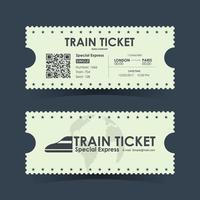The image displays a small, neatly-cut train ticket shown from both its front and back sides, set against a dark bluish-gray background. The ticket itself is white with detailed bluish-gray text and graphics. On the front, "Train Ticket" is prominently displayed in large letters in the middle, with "Special Express" underneath. To the left, there is an image of the front of a train, characterized by serrated edges. There is additional smaller text to the right that is unreadable due to the image’s size. The back of the ticket has "Train Ticket" centered at the top, with "Special Express" and a QR code on the left. The text also indicates a journey from London to Paris, but the rest of the text remains too small to decipher. The design is nostalgic, featuring embellishments and a possible watermark of a globe, adding to its vintage appearance despite the inclusion of modern elements like the QR code.